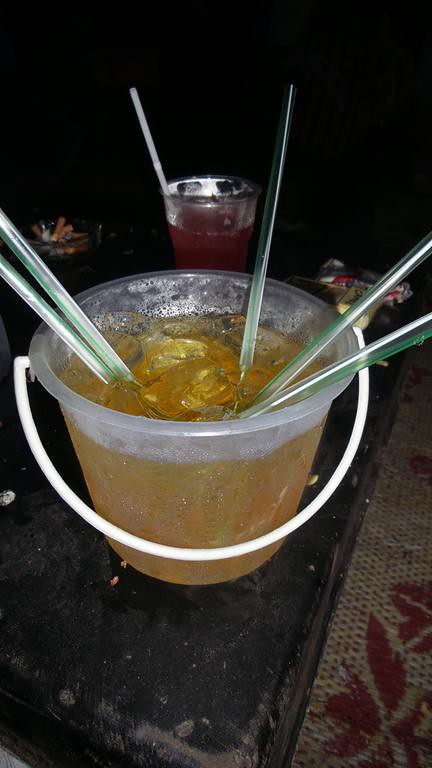In the photograph, a clear plastic bucket, resembling a child's beach bucket, takes center stage. It sits atop a black surface that appears to be a mat, which is itself resting on a beige rug adorned with red leaves. Inside the bucket is a golden-yellow gel-like substance mingled with ice cubes. Emerging from the bucket are several green and white straws. Positioned behind the bucket is a tall glass, three-quarters filled with a red liquid, with a white straw poking out from the left-hand side. The background is mostly dark, with indistinct objects barely visible beside the bucket, adding a sense of mystery to the scene.